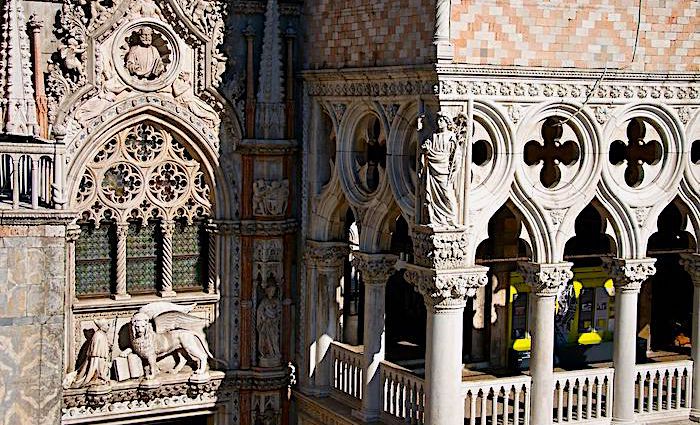The photograph showcases the grandiose architecture of the Ducal Palace in Venice, specifically its Porta Della Carta entrance, freshly conserved. The building, predominantly light brown and grey, is constructed from bricks that form patterns, with red and white elements adding color variations. Dominating the left side is an arched window topped with an elaborate statue of a man. Below this window, a detailed statue depicts a man facing a lion, adding to the narrative richness of the scene. The right side features an extravagant balcony supported by circular pillars that are adorned with a flower-shaped cut-out pattern at their tops. Further artistic details include cherubs climbing the stonework, contributing to the Flamboyant Venetian Gothic style. The entire facade is a marvel of intricate stone carvings and ornamental designs, embodying the historical opulence of the Ducal Palace. Additional decorations, possibly made of ceramic or clay, enhance the walls, inviting viewers to continuously discover new elements in the ornate craftsmanship.